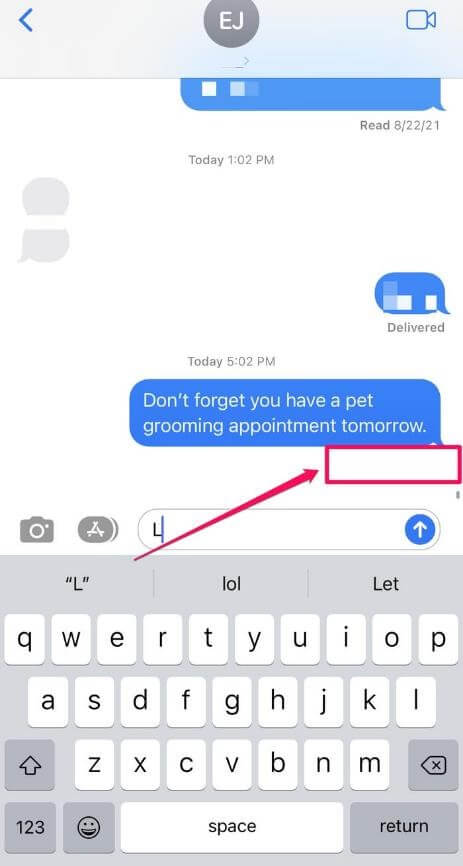Screenshot of a text conversation displayed on a cell phone screen. In the top left corner, there is a blue back arrow. The top bar features a very light blue, almost white, background. Centrally positioned within this top bar is a gray circle containing the white capital letters "EJ." To the upper right, icons for both camera and video functions are visible.

Below this header, the main screen transitions into the white backdrop of the text conversation itself. The initial blue text bubble near the top is partially cut off and redacted, but it's noted that it was read on August 22, 2021. Towards the bottom of the screen, timestamped "Today at 5:02 p.m.," the text bubble reads: "Don't forget you have a pet grooming appointment tomorrow."

Further down, there is some empty space followed by the input box where one would type a response. The overall layout is clean, though the incomplete and blurred details hint at privacy considerations.